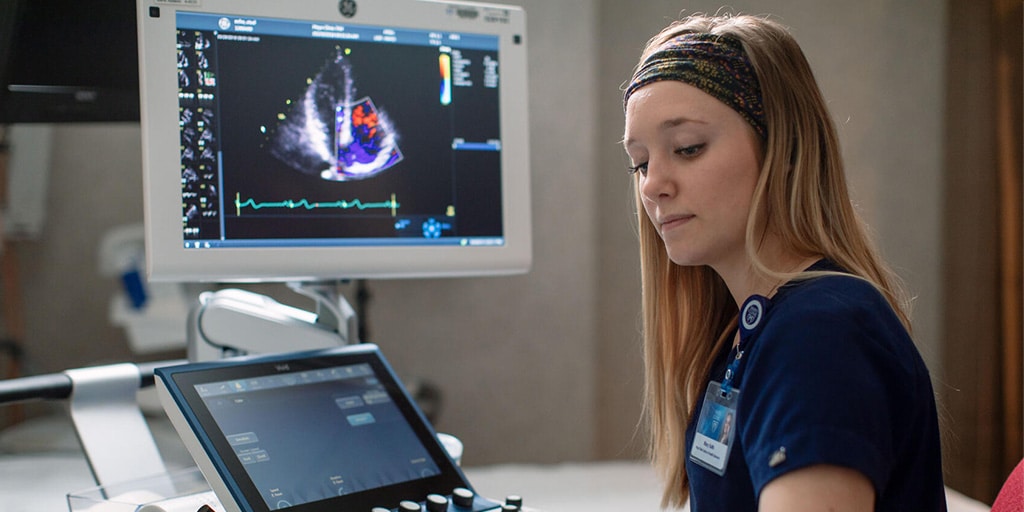In a well-equipped medical office room, a female technician in her late 20s or early 30s is captured in a moment of concentration. She dons navy blue scrubs adorned with a name badge, and her long blonde hair is partially covered by a stylish dark headband decorated with gold flowers. To her left, a monitor displays a detailed ultrasound scan, characterized by various colors including white, red, and blue. The ultrasound machine, positioned underneath the monitor, features several knobs and controls, suggesting she is adjusting these to fine-tune the scan. Her attention appears to be focused more on the adjustments rather than the screen itself.